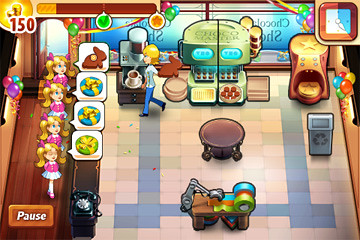This image is a screenshot from a vibrant and colorful mobile game, likely set in a bustling bakery or factory environment. The screen is filled with various interactive elements and a vivid display of details. In the top left corner, there's a gold counter showing the player has 150 gold. The top right features additional gold markers and a timer tracking the gameplay. The bottom left corner houses a pause button for stopping the game.

Central to the scene is a dynamic factory floor with several machines, including an espresso machine and a cupcake maker, surrounded by other equipment and furniture such as a table, a trash can, and a ribbon-cutting station. On the left side of the image, a woman is seen walking towards the counter, holding a chocolate bunny. Nearby, there is a group of identical little girls with two blonde pigtails, dressed in pink shirts with yellow and white skirts, eagerly placing their orders. The overall setting suggests a fast-paced, task-oriented game designed for mobile devices.